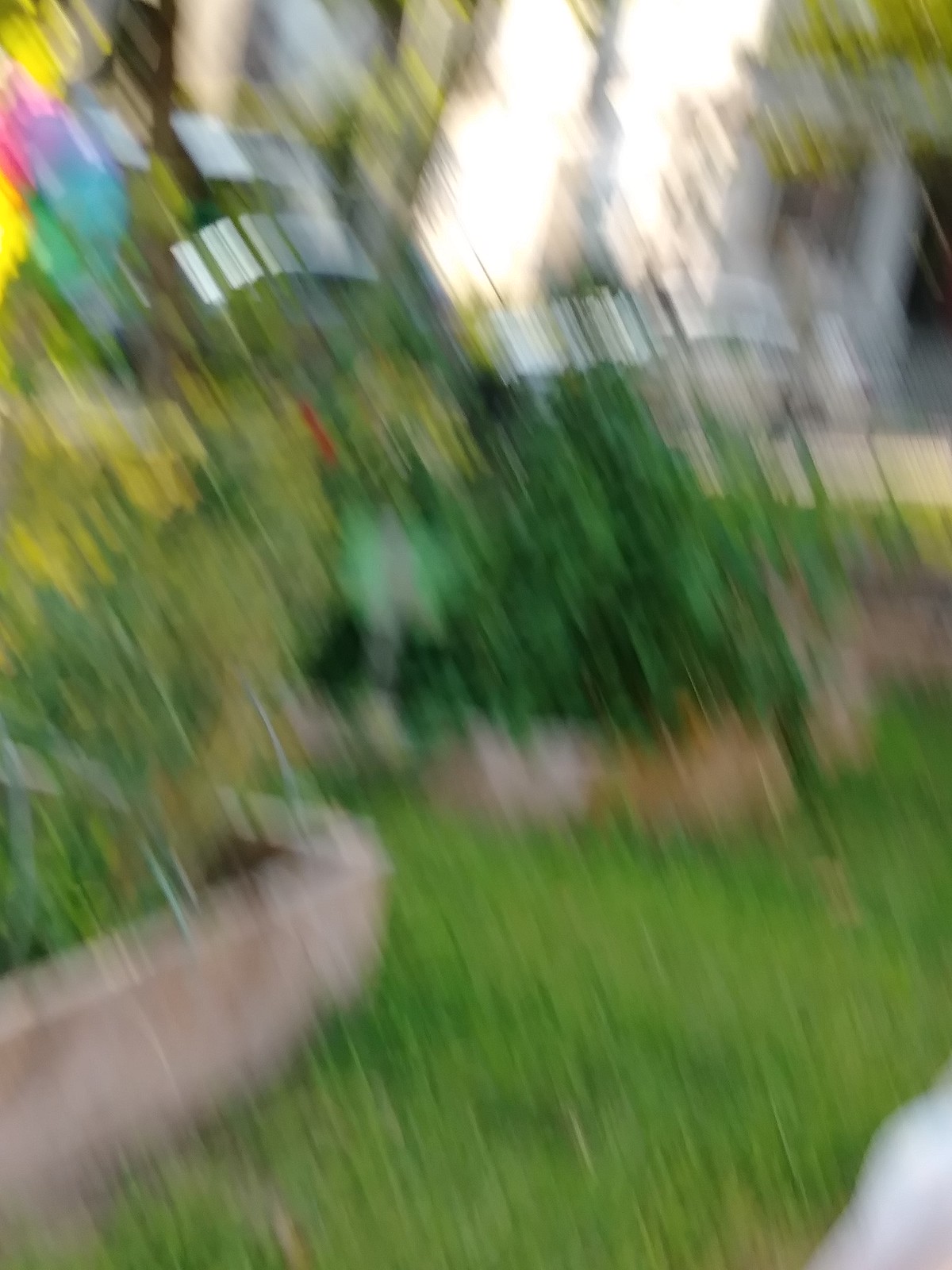A highly blurred photograph, possibly intentionally distorted for an artistic effect, captures a scene dominated by lush green grass and raised flower beds bordered in brown. The image appears to depict a rainfall, with water streaking diagonally from the left, adding to the blur. Despite the lack of clarity, vibrant colors pierce through the haze: splashes of yellow, blue, and pink intermingle towards the upper part of the scene. A peculiar silverish pattern or window-like structure spans the middle to the top of the photo, although its exact form remains indistinguishable due to the intense blurriness.